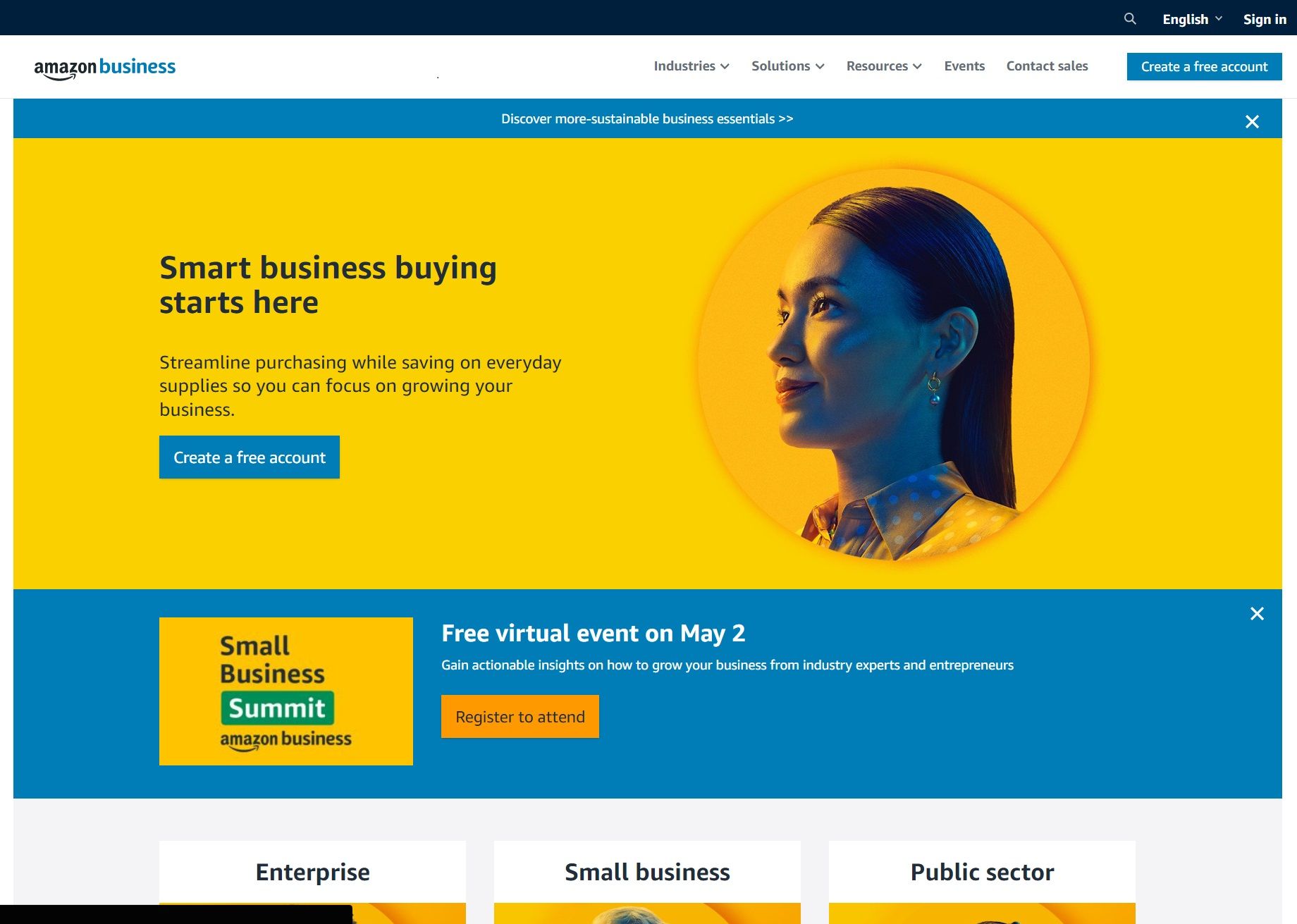This screenshot captures a horizontally structured webpage for Amazon Business. The prominent sections of the page are filled with blue and yellow hues. The header bar at the top is white, featuring a black top banner. On this header, a drop-down menu titled "Amazon Business" is positioned on the left, listing dropdown options such as Industries, Solutions, Resources, Events, and Contact Sales. Adjacent to this menu is a blue button labeled "Create a free account."

Beneath this header is a thin blue strip, followed by the main portion of the page, which boasts a bright black background. Central to this section is a circular inset photo of a woman with long black hair, dressed in a polka-dotted shirt, looking towards the left. Next to the photo, the text prominently reads "Smart Business Buying Starts Here," accompanied by additional descriptive text and another button that says "Create a free account."

The bottom section displays a blue banner with a yellow tab announcing the "Small Business Summit Amazon Business," touting a free virtual event on May 2nd, and features an inviting orange button labeled "Register to attend." The remaining part of the image includes three categories—Enterprise, Small Business, and Public Sector—from left to right. The bottom of the screenshot is truncated, cutting off any additional information.